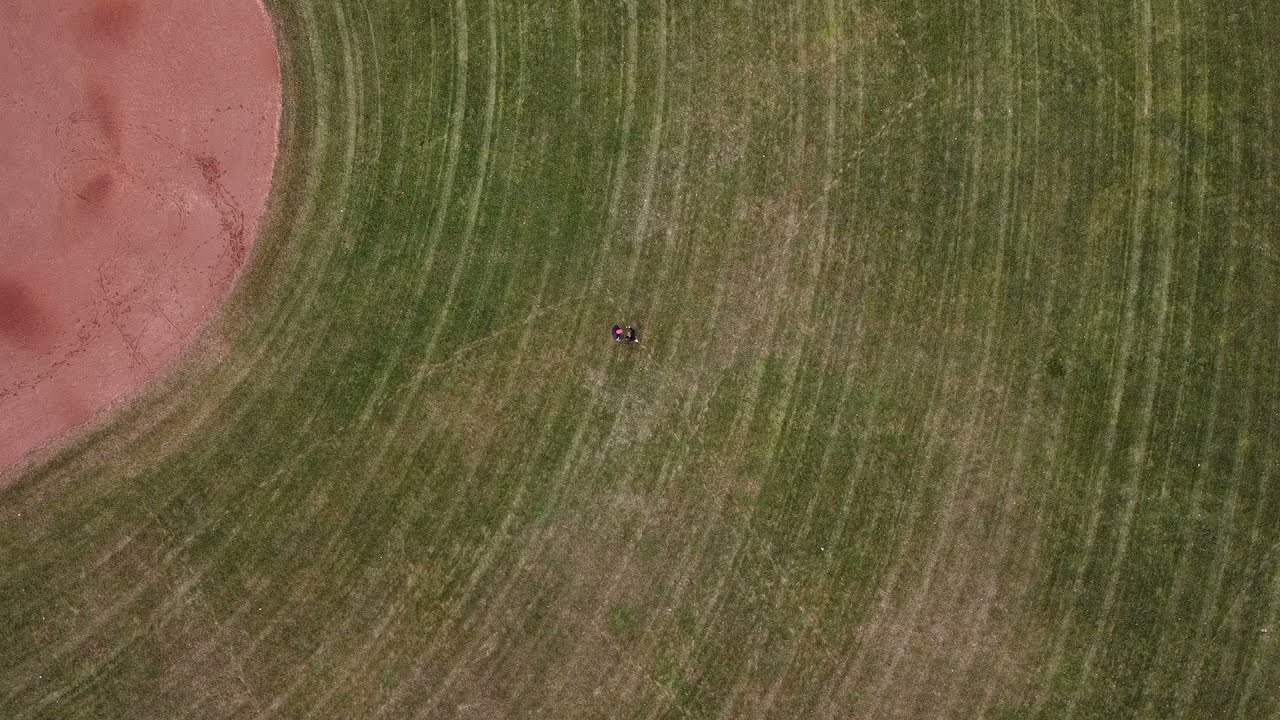The image is a top-down view of a mostly grassy landscape with distinct mowing lines curving in alignment with a circular dirt area located in the upper left-hand corner. The circular region of dirt, which could be a baseball field or similar open area, contrasts with the predominantly green terrain. The grass itself appears patchy, with some areas showing a tan color possibly due to dryness. In the center of the image, roughly 100 feet from the camera, is a person, likely on a ride-on lawnmower, contributing to the curved mowing patterns seen throughout the grass. The dirt area features a light red hue, with deeper red patches that might be wetter sections.